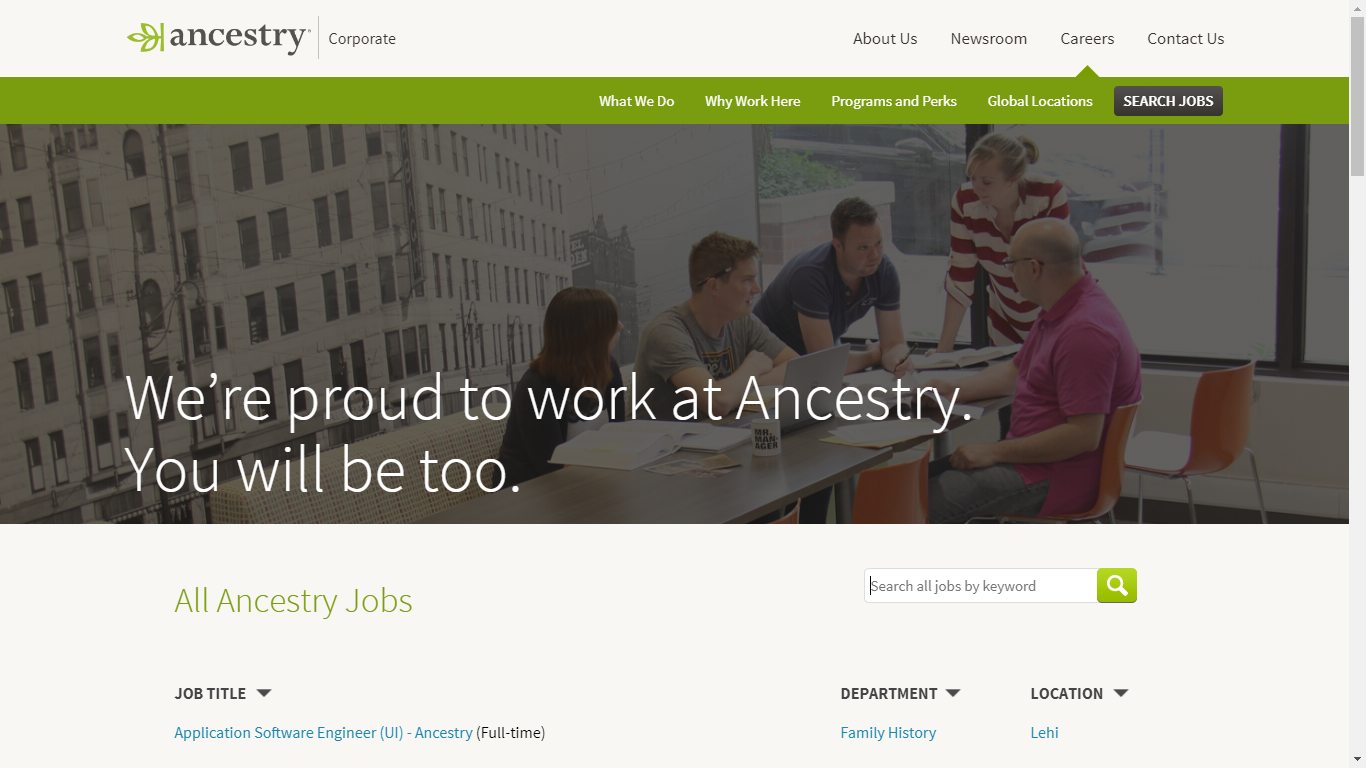This image is a screenshot taken from the website Ancestry.com. In the top left-hand corner, the Ancestry logo is prominently displayed. The top right-hand corner features a navigation bar with four links: "About Us," "Newsroom," "Careers," and "Contact Us." 

In the center of the image, there is a large, wide photograph depicting a group of people gathered around a table, indicating a social or casual work setting. On the table, there is a laptop and a collection of papers, suggesting a work-related meeting or collaborative session. The image is overlaid with the caption: "We're proud to work at Ancestry. You will be, too."

At the bottom left corner of the page, there is a link labeled "All Ancestry Jobs," suggesting that this section is geared towards job opportunities at Ancestry. In the bottom right corner, there is a small search bar with the prompt "Search All Jobs by Keyword," enabling users to search for specific job openings on the site.